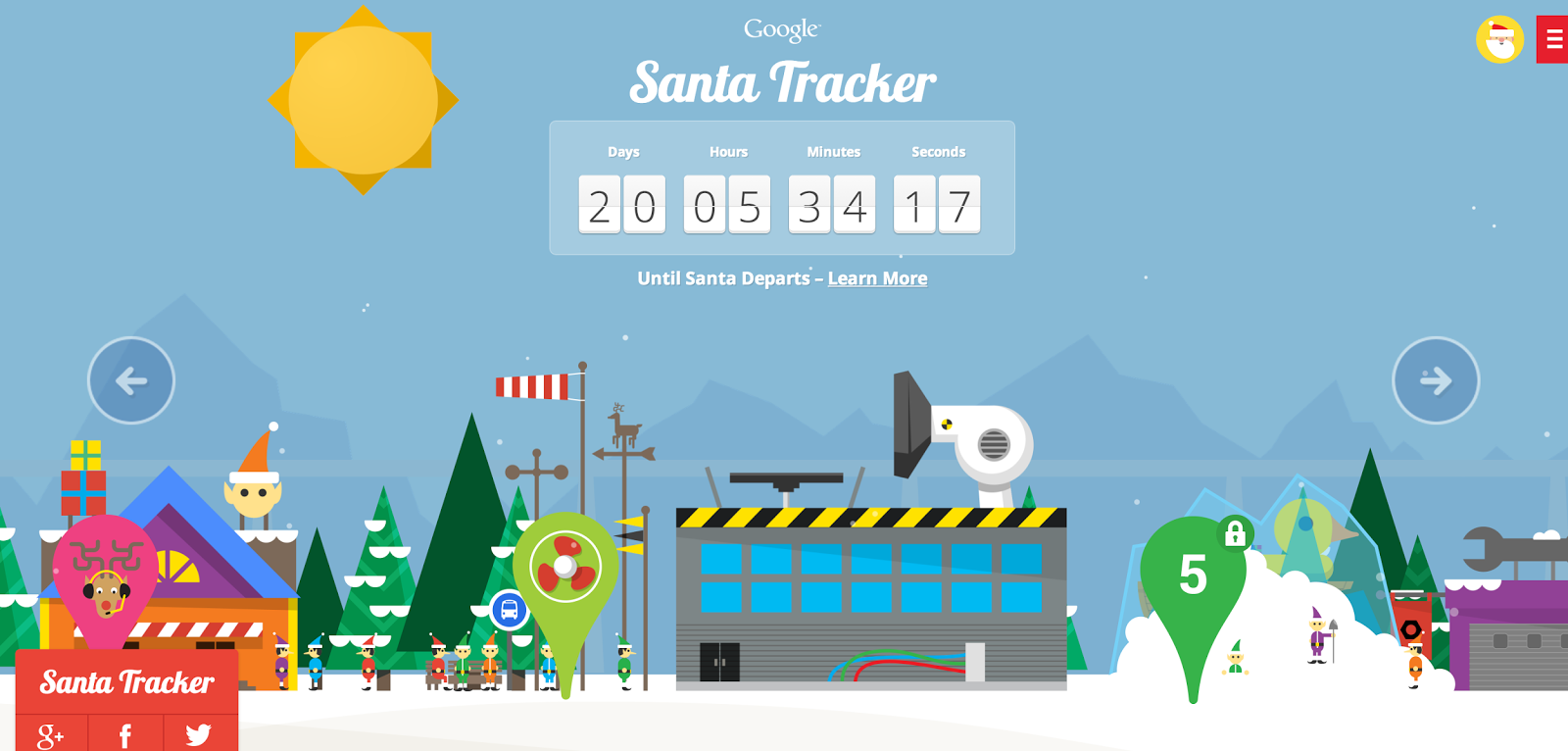The Google Santa Tracker image features a whimsical, cartoon-style scene set against a backdrop of a blue sky with the sun casting a cheerful glow. In the upper right-hand corner, Santa is depicted within a yellow circle, accompanied by a red box with vertical lines cascading down. The title "Google Santa Tracker" is prominently displayed in the top center of the image. A countdown bar, situated just below the title, indicates the time remaining until Santa departs: 20 days, 5 hours, 34 minutes, and 17 seconds.

The bottom left-hand corner of the image includes a small red box labeled "Santa Tracker." Social media icons for Google Plus, Facebook, and Twitter are neatly organized nearby. A reindeer, outfitted with headphones and a microphone, appears to be engaging in communication, adding a playful touch.

The lower half of the image showcases a bustling scene with various animated elements. A grey warehouse with black double doors is featured prominently, topped with a large hair-blower-like device and adjacent to a flag. Encased in ice, a duck adds a quirky element to the scene. A tool, resembling a wrench, is placed over a purple garage. Elves are seen standing and sitting in a snowbank, adding to the festive atmosphere. Navigation arrows on each side of the image suggest the ability to explore more of this imaginative Santa world. In the distance, mountains stretch across the horizon, completing this enchanting holiday setting.